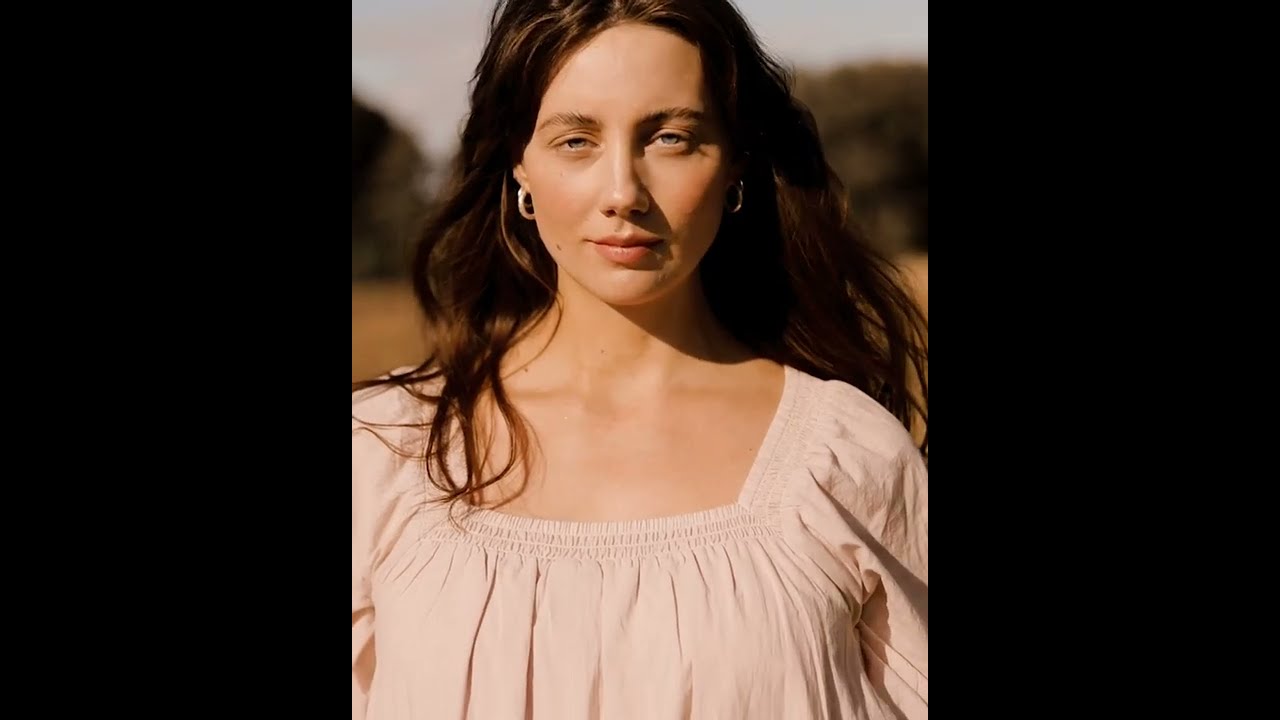The image depicts a young, fair-skinned Caucasian woman with long, flowing brown hair parted in the center. Her blue-gray eyes are barely open as she stares directly into the camera with a neutral expression. Her hair cascades past her shoulders, with the right side blowing slightly across her shoulder and the left side hanging straight down. She is adorned with hoop earrings, though the one on her right ear is obscured by shadows, while the shiny earring on her left ear is clearly visible.

She is wearing a peach-colored, wrinkled dress that features an elastic band over her shoulders extending across her chest. The material of the dress beneath the band is gathered in layered pleats. The background is out-of-focus, revealing a vague tree line with a blue sky above and a brown field below, suggesting a professional outdoor photoshoot.